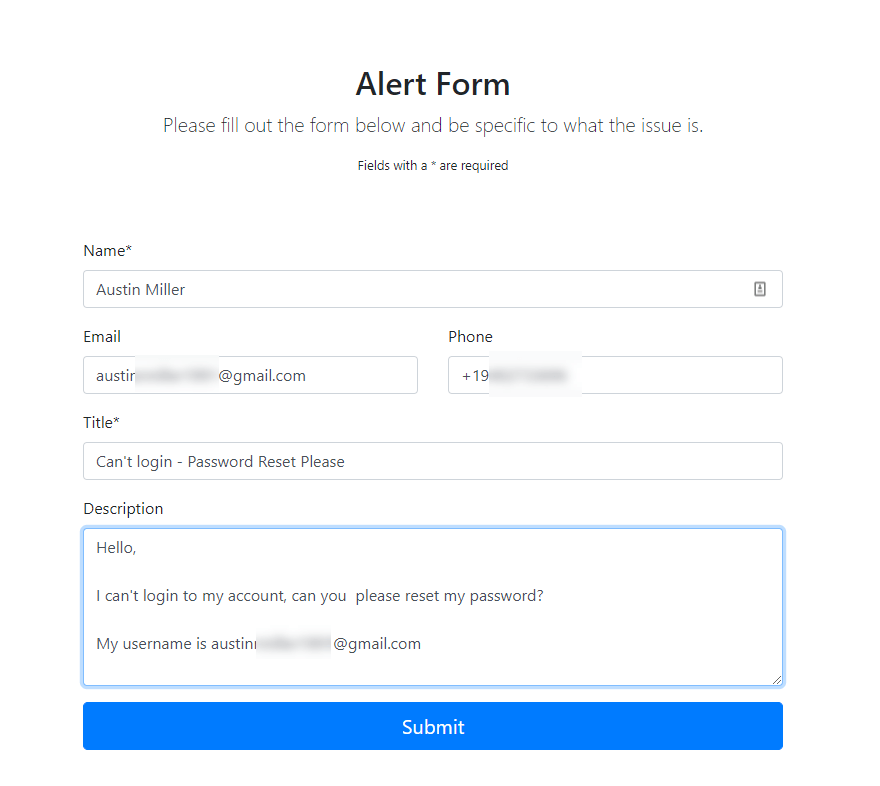This image, captured from a cell phone screen, displays an "Alert Form" page with a predominantly white background. Centered at the top, the text "Alert Form" is written in bold black letters. Below, a brief instruction reads, "Please fill out the form below and be specific to what the issue is," followed by a note indicating that fields marked with a star are mandatory.

The form begins with a field where the user, identified as Austin Miller, has input their name. Adjacent to this field is a download button. The next field contains Austin's email address, partially visible as "Austin…@gmail.com," with the rest blurred for privacy. Similarly, the phone number field shows only the initial "+19," with remaining digits obscured.

A mandatory field labeled "Title" states, "Can't log in, password reset please." In the "Description" section, Austin has typed a message requesting assistance: "Hello, I can't log into my account. Can you please reset my password?" This is followed by the partially blurred username, "Austin…@gmail.com," again protected for privacy. The description area and the long "Submit" button are highlighted in blue, emphasizing their importance in the form submission process.